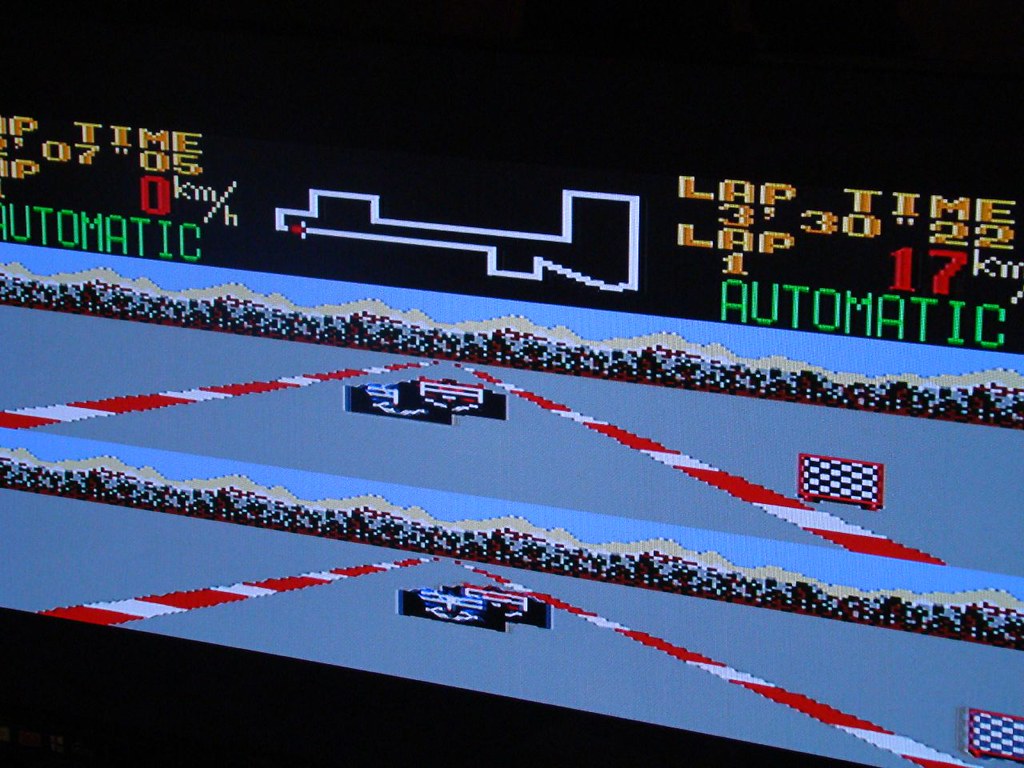The image is a detailed screenshot of an old-school, low-resolution video game, likely a racing game given the described elements. It features a dual-player split-screen layout, with each player's section showing a racetrack from a top-down perspective. The tracks are bordered by red and white bumper stripes, which are more prominent in the upper player’s screen. The lower part of the track hosts two pixelated race cars—one blue and one red—amid simplified tree representations. The background of both sections showcases a mountain range capped with white snow under a blue sky. 

Above both racing tracks, the Heads-Up Display (HUD) shows crucial game information. This includes "laps" and "times" in black text, with "automatic" written in green, and a white outline map of the racetrack. Additionally, the HUD displays a lap time of "3:30.22," underlined by a lap count "17 kilometers." Notably, a simplistic, boxy creature-like symbol is centered in the upper HUD area. The game’s graphics are highly pixelated, emphasizing its retro, low-bit aesthetic.